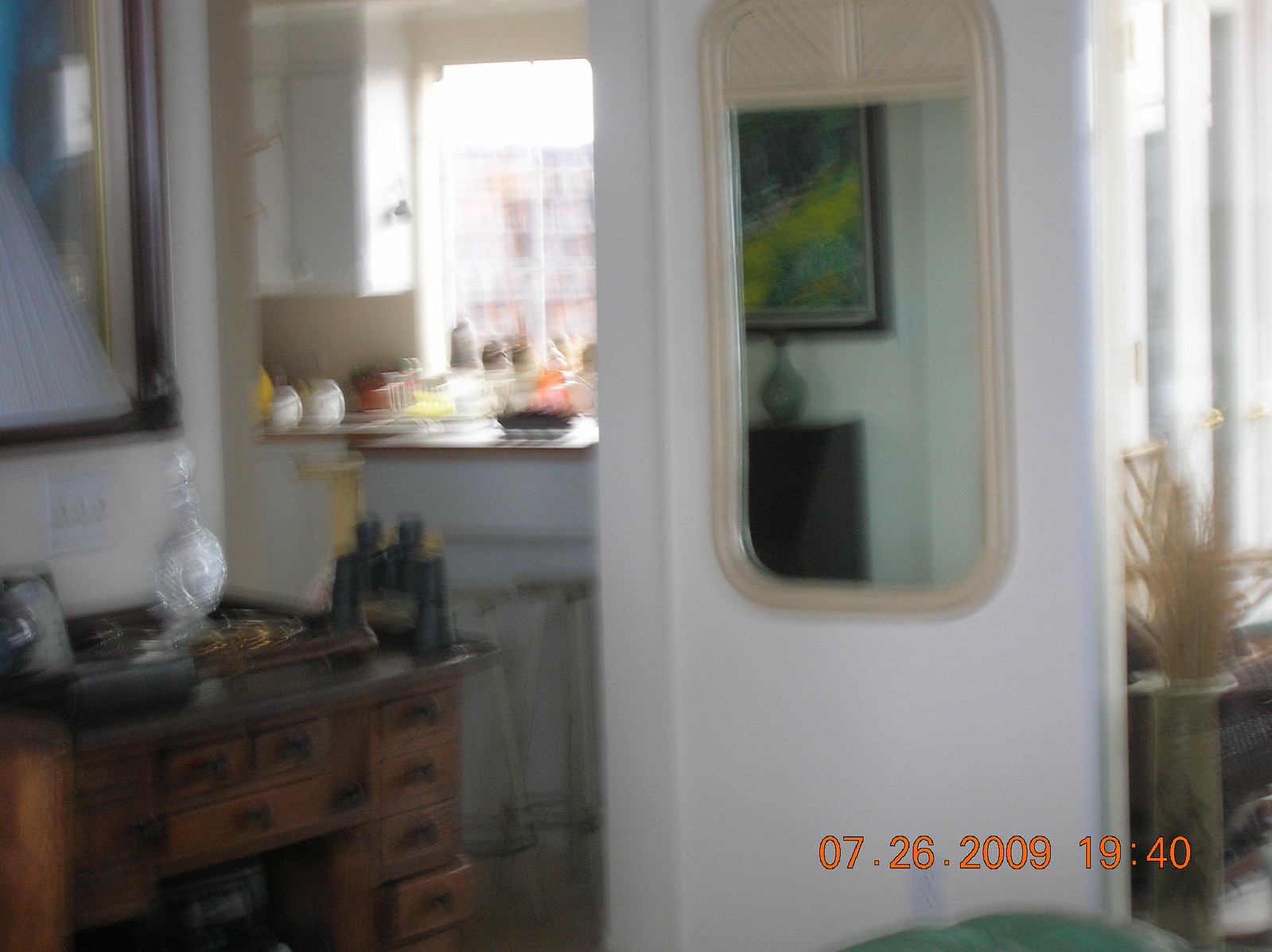In this slightly distorted photograph taken indoors on July 26, 2009 at 19:40, a cozy section of an apartment or living room is captured in detail. The scene reveals a blend of a kitchen and a study nook. The kitchen, located towards the back, features a white wall, white cabinets, a window with sunlight filtering through, and a counter cluttered with dishes and various items. Tall stools are placed in front of a ledge with additional kitchenware.

Up close, a dark brown wooden study desk with an old-fashioned charm dominates the area. On top of the desk, a pair of black binoculars, a white crystal urn possibly filled with alcohol, and a clear glass vase sit prominently. The desk is equipped with multiple small drawers and shelves; specifically, four on the right and three in the center. A large mirror with a brown trim is mounted above, reflecting a wall picture framed in dark brown, featuring green and blue hues.

To the right of the desk, a white door with a long mirror framed in beige wood and a rattan-like top stands in view. The mirror also reflects more room details, including a brown cabinet topped with a vase. Further to the right, a room with white curtains and a beige planter—possibly containing a fern—is visible. The timestamp "07-26-2009-1940" is clearly marked in orange at the lower right-hand corner of the image.